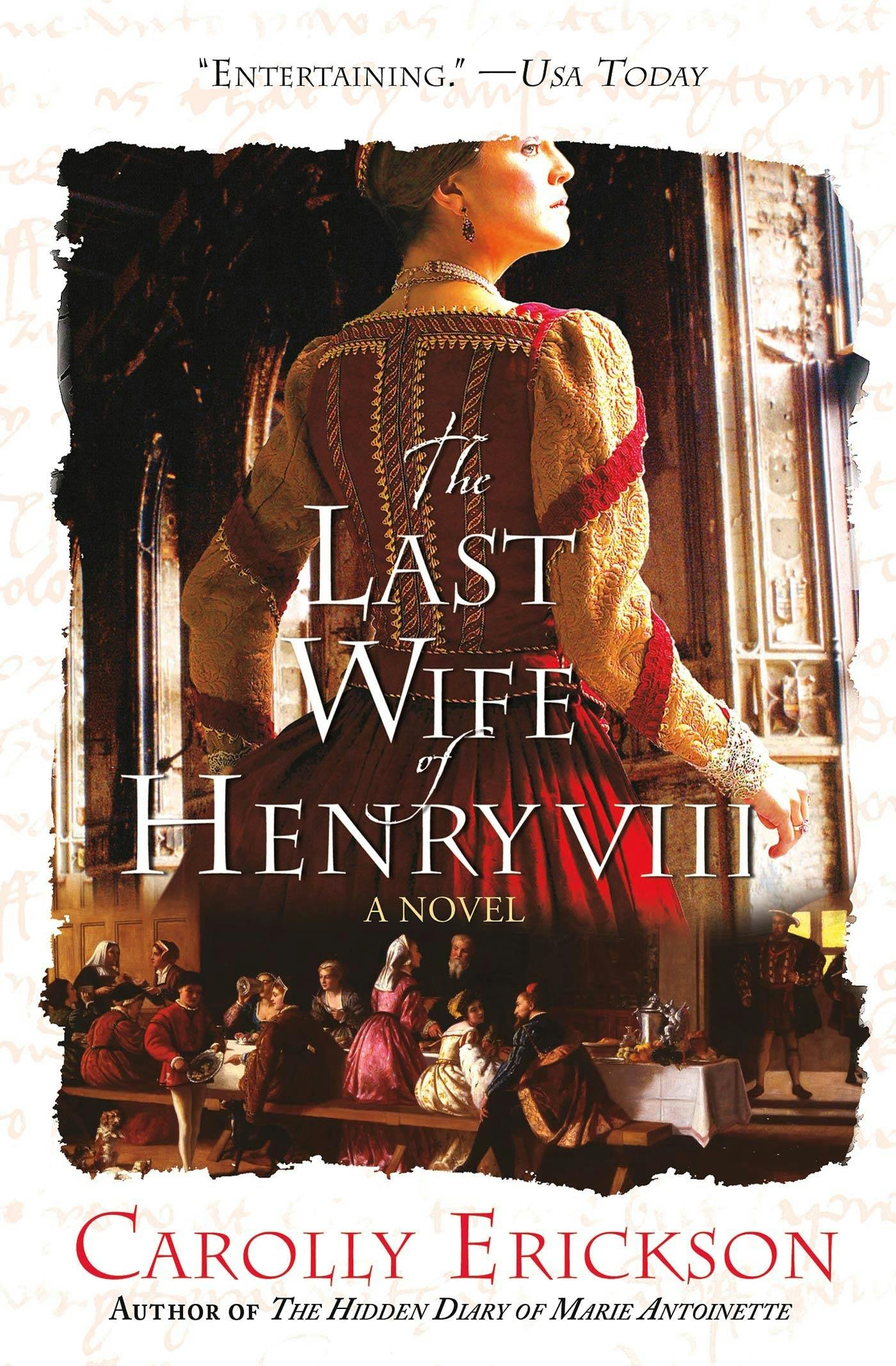The image is a vertically aligned rectangular book cover of "The Last Wife of Henry VIII" by Carolee Erickson. The title, rendered in large white all-caps, dominates the middle of the cover with "A Novel" in smaller yellow all-caps beneath it. At the very top, in parentheses, is the quote "Entertaining" attributed to USA Today. The author's name, in red all-caps, appears at the bottom, followed by the subtitle "author of The Hidden Diary of Marie Antoinette" in smaller black font. 

The main image portrays a close-up of a regal woman from the back, clad in a sumptuous gold and red long-sleeve dress with red ruffled skirts. She is adorned with a pearl necklace and has her head tilted slightly to the right. The background features a room filled with people in elaborate gowns, with men in red coats, suggesting a royal setting or a grand celebration. The detailed illustration captures the historical and royal essence of the book's subject.